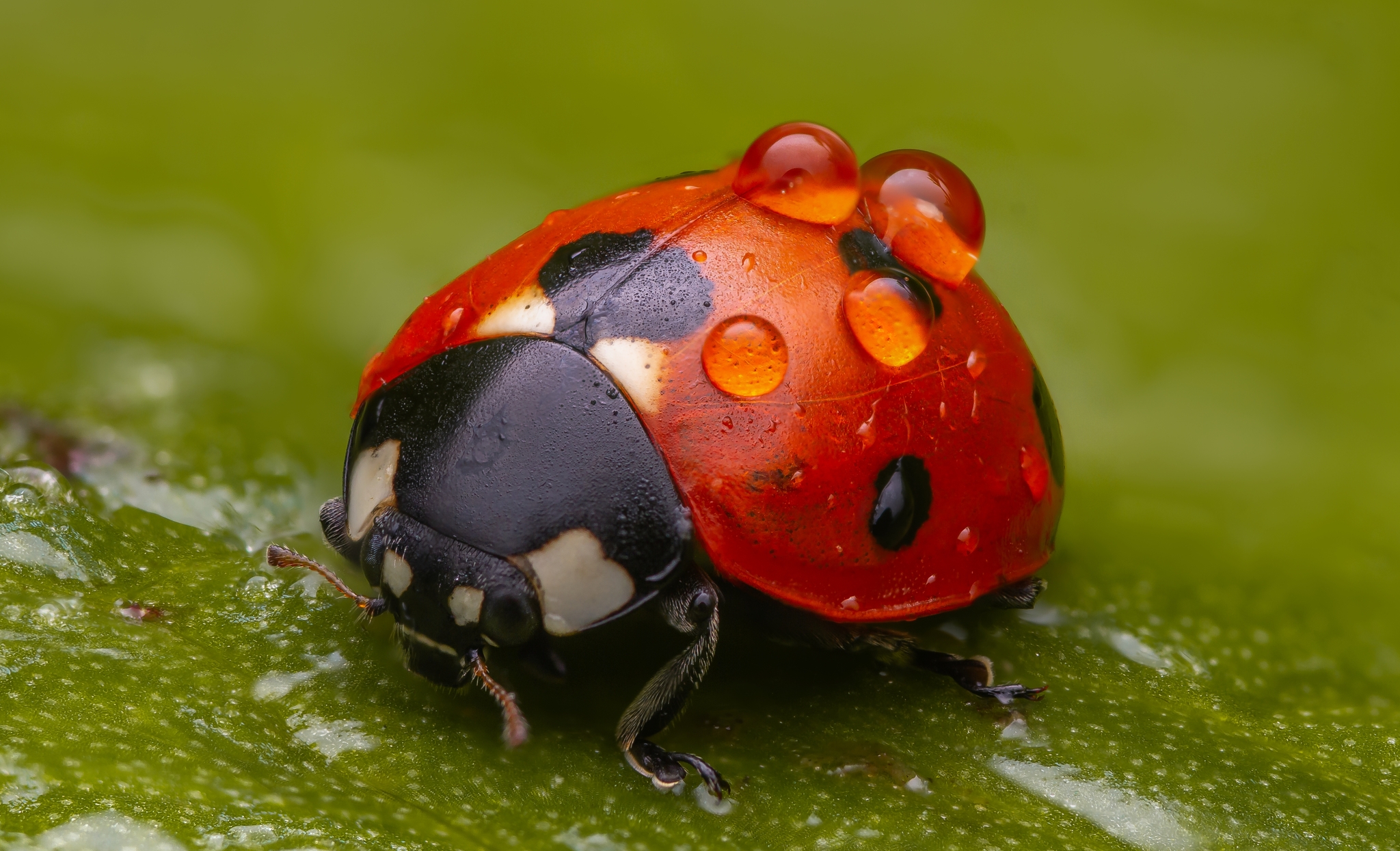This is an incredibly detailed macro shot of a ladybug, facing left and perched on a dew-covered leaf. The background is an olive green that becomes more textured and white-spotted towards the bottom, although it remains entirely blurred out. In sharp contrast, the ladybug and the leaf it rests on are vividly clear. The ladybug's bright, reddy-orange back is adorned with four black spots and two large white dots near its head, transitioning into the darkness of its black head where you can also see intricate details like the antennae and multiple droplets of water. Specifically, four large droplets of water sit on its hard, shiny shell, reflecting the red color of the ladybug itself. Visible are three of the ladybug's legs and part of another, contributing to the overall fascinating close-up that reveals its minute details.